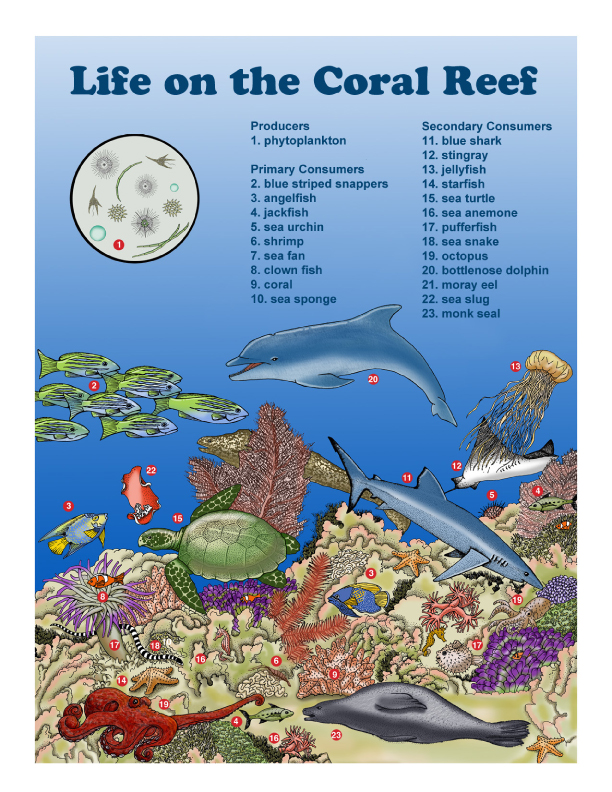The poster, set against a blue background, is titled "Life on the Coral Reef" at the top. It features a detailed depiction of various marine life, showcasing both producers and secondary consumers. The producers, listed from 1 to 10, include phytoplankton, blue-striped snappers, angelfish, jackfish, sea urchin, shrimp, sea fan, clownfish, coral, and sea sponge. Below them, the secondary consumers are displayed, such as blue sharks, stingrays, jellyfish, starfish, sea turtles, sea anemones, pufferfish, sea snakes, octopuses, bottlenose dolphins, moray eels, sea slugs, and monk seals. The creatures are illustrated swimming in the water with the ocean floor visible at the bottom of the image. The setting is bright and clear, with abundant lighting highlighting each organism. Every picture is labeled, and a chart at the top categorizes them, contributing to the educational value of the poster.